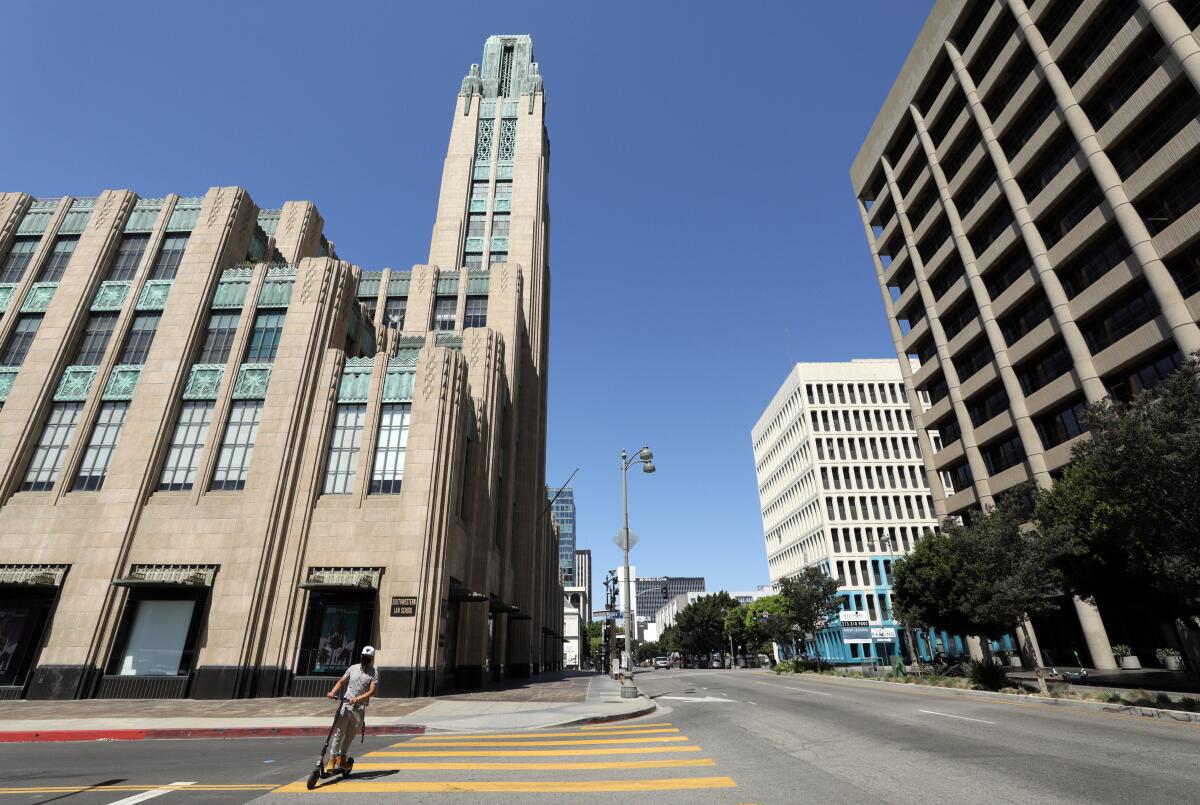The image captures a bustling urban setting in an American downtown area, showcasing distinct architectural styles and open spaces. Dominating the right side of the scene is an immense, 10-story parking structure, reminiscent of those found near major attractions like Disneyland. Opposite this, on the left side, stands a striking post-modern building featuring layered facades and a central tower. The central viewpoint highlights a man in a short-sleeved gray t-shirt and a baseball cap, riding an electric scooter across a yellow-striped pedestrian crosswalk. The street is notably devoid of cars or other pedestrians, save for a single distant vehicle. The backdrop includes a variety of buildings, some with blue-tinted windows and others with a pristine white exterior, while a few leafy dark green trees provide a touch of nature amidst the concrete. Under a clear, cloudless sky, the scene is illuminated by bright daylight, enhancing the visibility of every element, including a nearby lamp post with dual lights.